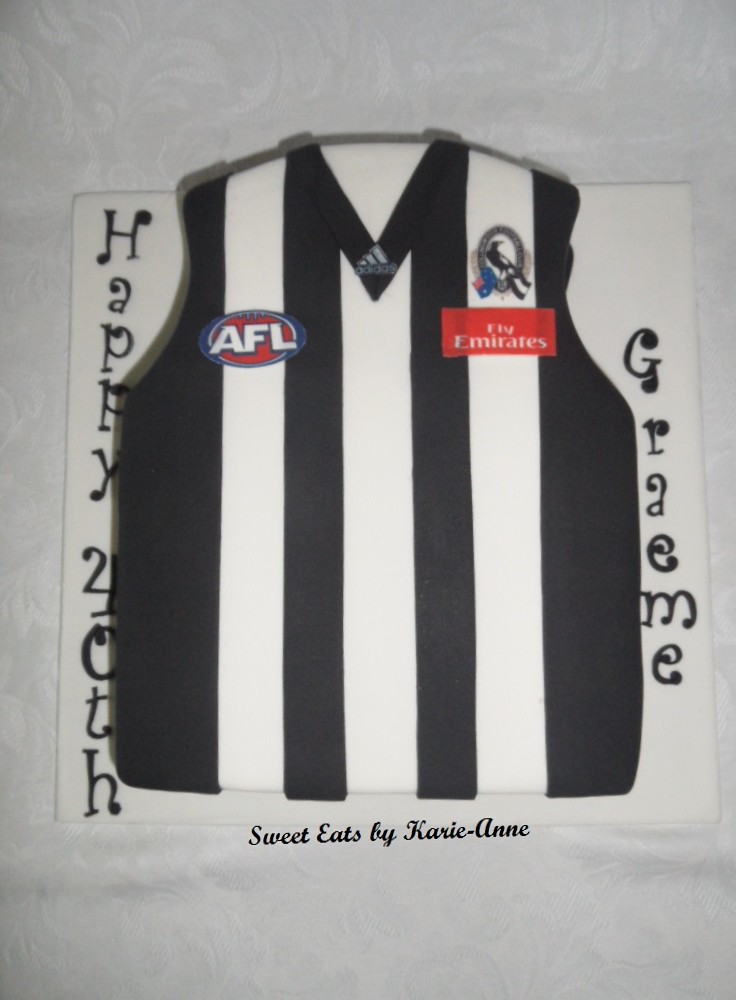This vertical rectangular image showcases a detailed cake designed to resemble a referee's uniform. The cake features distinctive vertical black and white stripes, mimicking the look of a short-sleeve vest. On the right chest area of the cake, a white block letter "AFL" insignia is visible, similar to a name tag. Toward the left chest area, a rectangular red name tag reads "Fly Emirates" in white letters. A sterling silver circle with a blackbird standing inside it is situated above the "Fly Emirates" tag. The cake sits atop a white textured background or possibly a piece of paper or poster board. Vertically inscribed along the left side of the background are the words "Happy 20th," while the right side reads "Graeme," with letters stacked on top of one another. Below the cake, it reads "Sweet Eats by Carrie Ann," indicating the creator of this celebratory confection. The setting appears indoors, suggesting a festive occasion, possibly commemorating Graeme's 20th milestone.